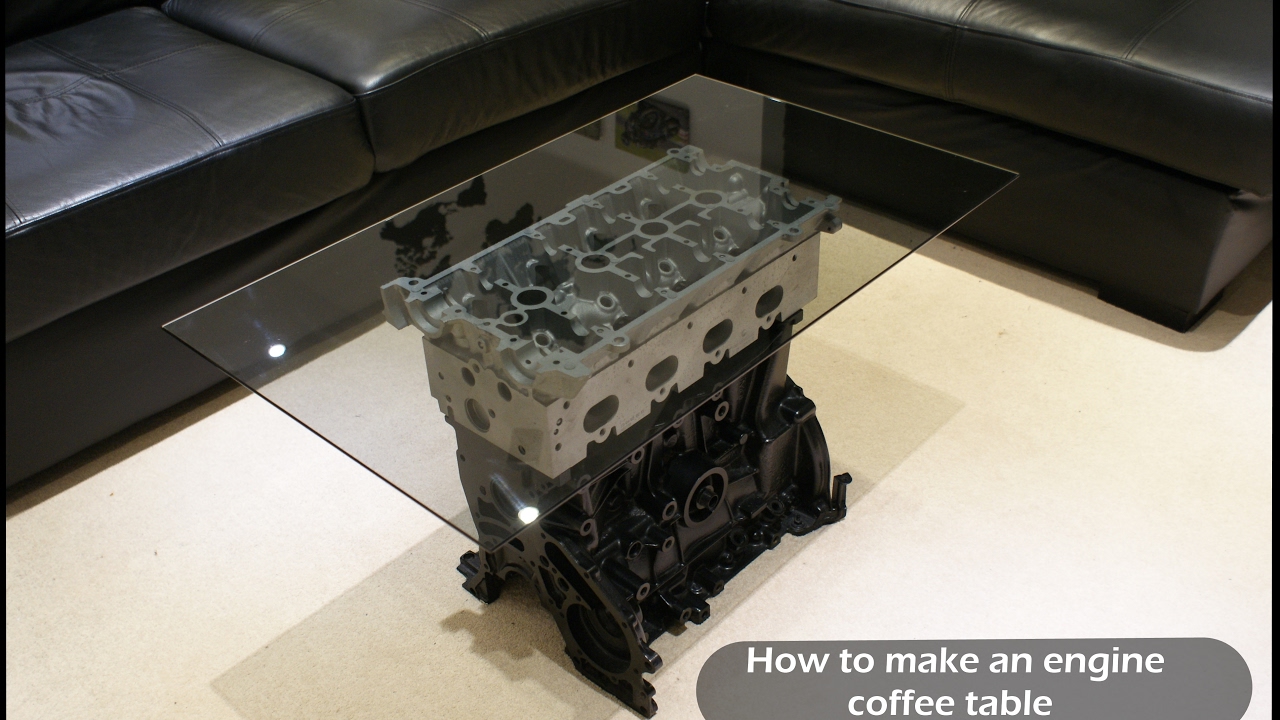The horizontally aligned rectangular image features a well-illuminated living or family room with a light beige tiled floor. In the background, there's a dark brown leather L-shaped sectional sofa, stretching from the upper left to the upper right of the image, with visible shadows and light reflections. A noticeable mark on the top left of the sofa suggests recent use.

Centered in the foreground, a distinctive coffee table stands out. Its base resembles a car engine, constructed with a black bottom and a gray top, appearing as though it's made out of Legos. Atop this engine-like base is a flat pane of glass that reflects the light from the room. The coffee table casts a shadow beneath it, emphasizing its presence. In the lower right corner of the image, white text against a taupe-colored oval background reads, "How to make an engine coffee table."